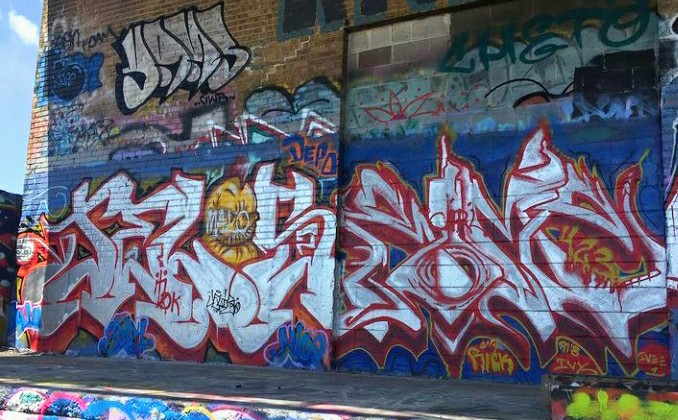The vibrant photograph captures the side of an abandoned brick building adorned with extensive layers of graffiti. The original brown brick is barely visible at the top of the image, hinting at the building's past before it was overtaken by urban art. The majority of the wall features a blue background that appears to cover older graffiti, with multiple layers and overlapping pieces suggestive of numerous contributions over time. Dominating the scene is a large mural consisting of squiggly white text outlined in red, adding a dynamic feel to the composition.

A striking, yellow rubber duck with a mohawk is prominently positioned on the middle left, serving as a whimsical focal point. Interspersed amongst the graffiti are red letter notes, including the sequence "4, 2, 3," and signatures such as "Rick" and "Ivy" written in yellow towards the bottom. Various other elements, like white letters outlined in black, can be seen blending with the remaining visible brickwork at the top.

The artwork extends down to the sidewalk, with further graffiti stretching along the edge of the curb and on an object in the lower right corner. Overall, the image captures a layered, chaotic, yet intriguingly colorful testament to urban expression and creativity.